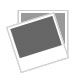The image showcases an old, intricately designed smoking pipe resting within an open, vintage-style case. The case, which appears to be made of brown wood or leather with a small gold clasp and tarnished gold hinges, is opened to reveal a cream-colored, furry interior, possibly velvet. The pipe itself is positioned towards the bottom center of the vertically rectangular frame and is shaped like a human hand holding the pipe bowl, with detailed carvings that have worn patches, revealing tan spots. The bowl is light brown, while the pipe stem is shiny and darker brown, curving elegantly. An insignia is visible on the interior of the case, which also contains some worn, hard-to-read text that includes the word "genuine." The photograph is taken indoors on a table, emphasizing the antique and well-preserved nature of the smoking pipe and its ornate case.